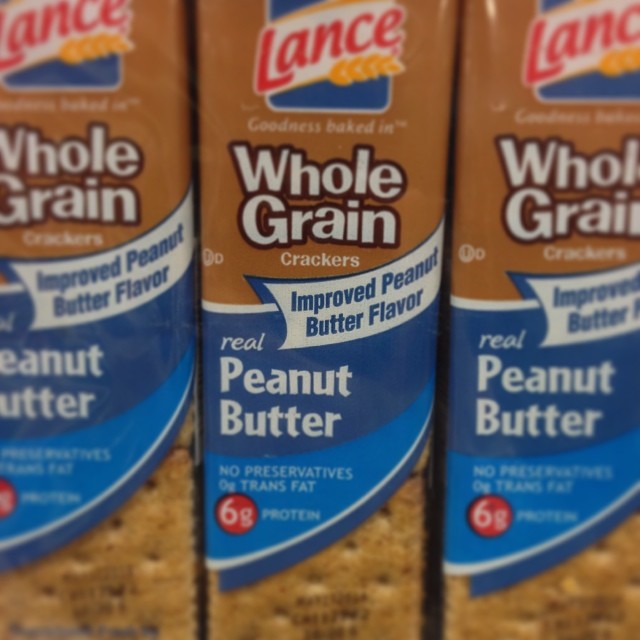The close-up photo showcases three packages of Lance Whole Grain Crackers. Each package prominently displays the Lance brand logo, adorned with a golden sheaf of wheat beneath the name. Above the main product name, "Whole Grain Crackers," a small text reads "Goodness Baked In". Below "Whole Grain Crackers," a label highlights an "Improved Peanut Butter Flavor." Further down, a blue banner states "Real Peanut Butter" in white text, accompanied by additional details: "No Preservatives," "Zero Grams Trans Fat," and "Six Grams of Protein," with the "Six Grams" highlighted in a red circle for emphasis. The transparent section at the bottom of the packaging provides a glimpse of the crackers themselves, revealing their toasty brown color.